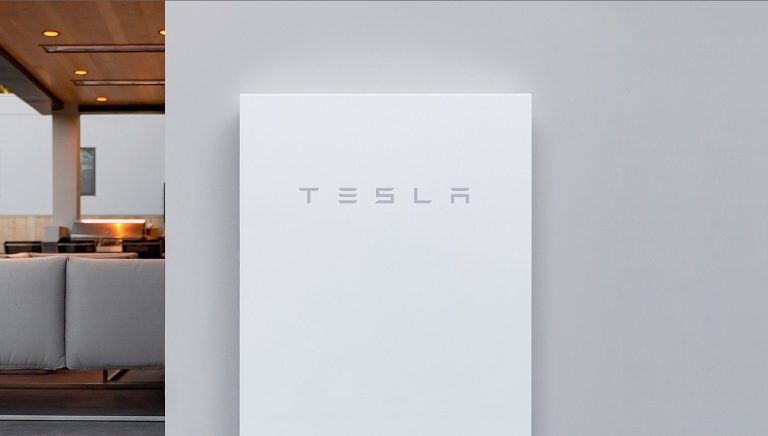This image showcases the left side of a room, prominently featuring a column or section resembling part of a house. To the left, gray chairs styled like a couch are positioned beneath a wooden roof alcove, giving the appearance of an indoor-outdoor patio area. A white wall serves as a backdrop, partially adorned with a framed painting. Below the pillar supporting the canopy structure, there is a stainless steel grill or cooking device, slightly obscured in the background. On the right side of the image, a stark white wall stretches into view, with a small white square centered on it, displaying the word "Tesla" in the company's distinctive font and logo.